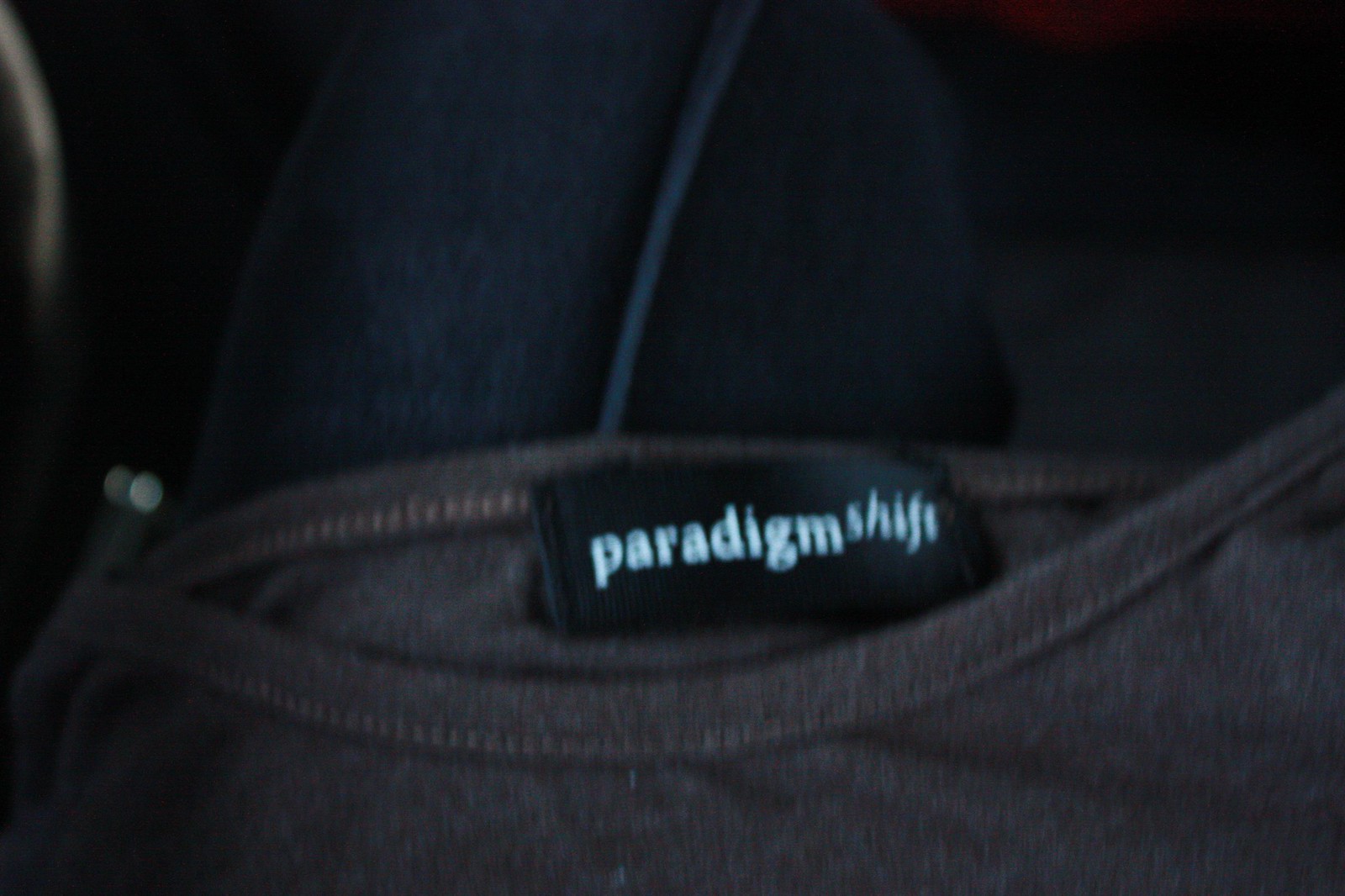This image shows a detailed close-up of a dark gray shirt draped over someone's blue jeans-clad lap. The shirt features a black rectangular tag that reads "Paradigm Shift," with "Paradigm" in white bold text and "Shift" in italics. The poor lighting in the photograph makes it challenging to determine the exact color of the shirt, which could also be dark brown. Only the neck part of the shirt is visible, revealing stitching around its wide, cut-out collar. Additionally, a cord runs down the side of the person's blue jeans, identifiable by a sewn-in seam. Although the carpet is obscured, it appears to be a dark color, hinted at by the limited light cast in the scene. The overall image is somewhat blurry, further complicated by the dark and shadowy background.